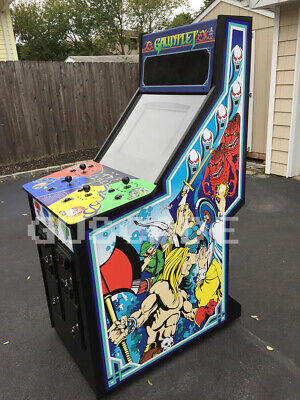This photograph captures a vintage standalone arcade game called "Gauntlet" set up in someone’s driveway, possibly for sale or display. The scene is framed by a six-foot tall brown wooden fence in the distance and a portion of a beige-shingled house with white trim on the right, including a view of the garage. The Gauntlet arcade game, with its screen currently off and showing white, prominently features its title in green lettering across the top. It is designed to accommodate four players, each with their own joystick in red, blue, yellow, and green. The front panel includes coin slots, and the side of the cabinet is adorned with colorful, cartoon-style artwork depicting the game’s characters—a blonde, shirtless hero wielding an axe, surrounded by a variety of foes in red, yellow, green, blue, white, and black.